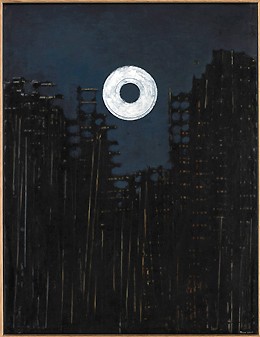The image appears to be a complex night scene, depicting abstract elements that evoke a surreal landscape. Dominated by a black background, the painting features a perfectly circular white object resembling a donut or a bright moon with a central hole, allowing the dark sky to peek through; this adds an impression of a solar or lunar eclipse. This circular formation is positioned roughly two-thirds of the way up the image, anchoring the composition. Branching from the lower sections toward the middle, intricately interconnected structures resemble thin, black pipes or densely populated tree trunks with silver, lightened extensions reaching upwards and pointing to the right. These metallic-like formations vary in height; some rise three-quarters up the page while others only extend halfway, creating a layered and textured visual effect that suggests a mysterious, industrial, or forested environment. The background transitions to a navy blue sky interspersed with lighter patches, providing depth and furthering the nocturnal, enigmatic atmosphere.